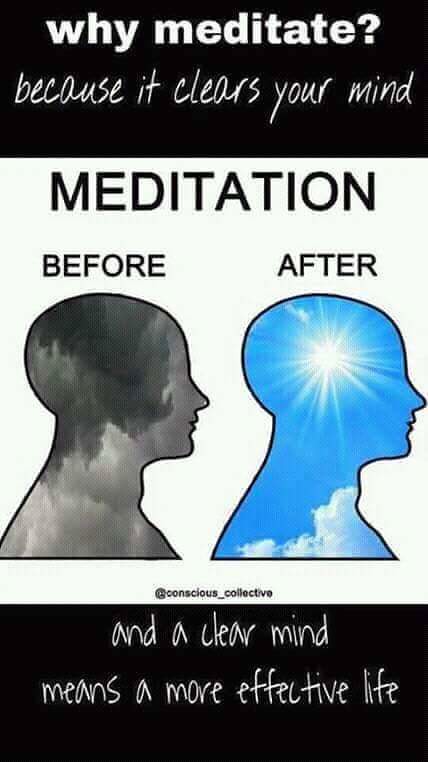The poster, designed to promote meditation, is divided into three distinct sections with a black-white-black color scheme. The top third features a black rectangle with white lowercase lettering that poses the question, "why meditate?" followed by the answer, "because it clears your mind." 

The middle section has a white background and prominently displays the word "meditation" in black lettering, followed by a "before and after" illustration. On the left, a drawing of a human head depicts a gloomy, cloudy, and dark state labeled "before." On the right, another human head illustration is filled with bright, sunny skies and white fluffy clouds, labeled "after."

The bottom section returns to a black background with white lowercase text, stating, "and a clear mind means a more effective life." The concise imagery and consistent color scheme work together to emphasize the benefits of meditation in achieving a clear and effective mind.